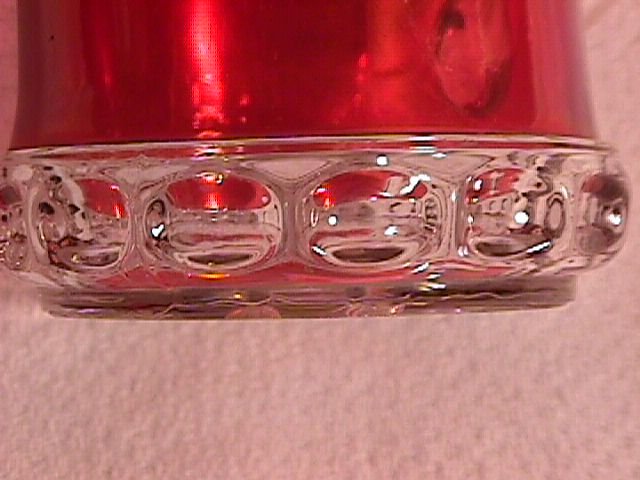This image showcases a close-up of the ornate bottom section of a ruby-red, early-pressed glass mug. The glass base reveals intricate detailing, including four cut circles and bubbles within the glass. The vivid ruby-red portion of the mug contrasts with the clear glass base. The mug rests on a white, woven-patterned tablecloth, adding texture to the otherwise simple background. The exact context of the mug's size remains ambiguous, though its reflective surface and detailed craftsmanship suggest it is a piece of dishware or decorative glassware.